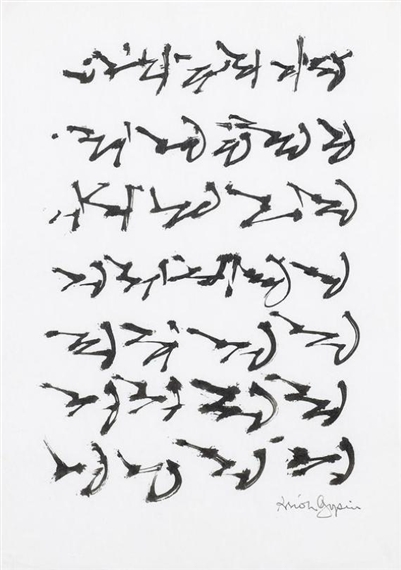The image depicts a modern painting featuring seven rows of handwritten black characters on a slightly off-white background. Each row contains a varying number of characters, written in an unrecognizable, asymmetrical script that resembles Asian writing but more closely resembles zigzags or child's scribbles. The characters are thick and evenly spaced, with each row maintaining a neat and orderly appearance. The first row has three characters, the second has five, the third has four, the fourth has two larger characters centered, and the remaining three rows each contain four characters. In the lower right corner, there is an artist's signature in freehand, reading "Armand Gasperin," written in a lighter shade of black. The overall aesthetic is that of ink sketches painted with a magic marker against the white background.